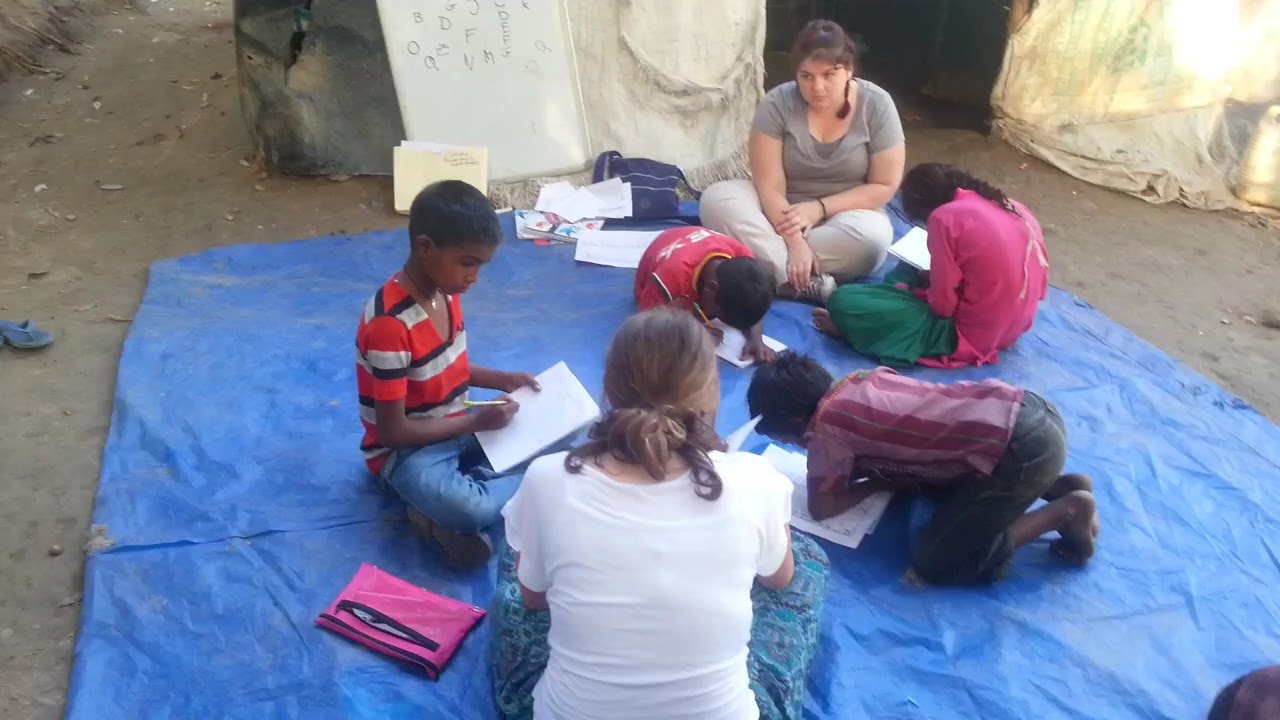In this detailed photograph, six individuals are gathered outdoors on a large blue tarp that stretches across dirt terrain, suggesting an excavation or field trip setting. The group comprises two European-looking women and four Indian children, creating a diverse mix. The tarp is positioned centrally, surrounded by scattered rubble and dirt, indicating a rough, possibly developing area. 

One of the women, seated at the far end, faces the camera wearing a gray top and white pants. A blue bag and some papers, as well as a tan folder, rest beside her on the dirt. Opposite her, a woman with her back turned towards the camera wears a white shirt and bluish pants, her brown hair tied back. 

Among the children, a boy in a red top faces slightly towards the camera, intently writing on a paper. To his right, a girl in a pink top and green pants also writes, facing away from the camera. Another child, a boy in dark shorts and a vertically striped pink shirt, kneels on the tarp, focused on his papers. Beside him, another boy in a horizontally striped red shirt with blue shorts writes diligently. 

In the background, a whiteboard with alphabet letters like "A" and "D" hints at a learning activity. The surrounding scenery includes white and brown stone formations, further emphasizing the rugged, outdoor environment. The setting suggests a field school or perhaps a missionary teaching scenario, highlighting the collaborative effort in education despite the challenging conditions.